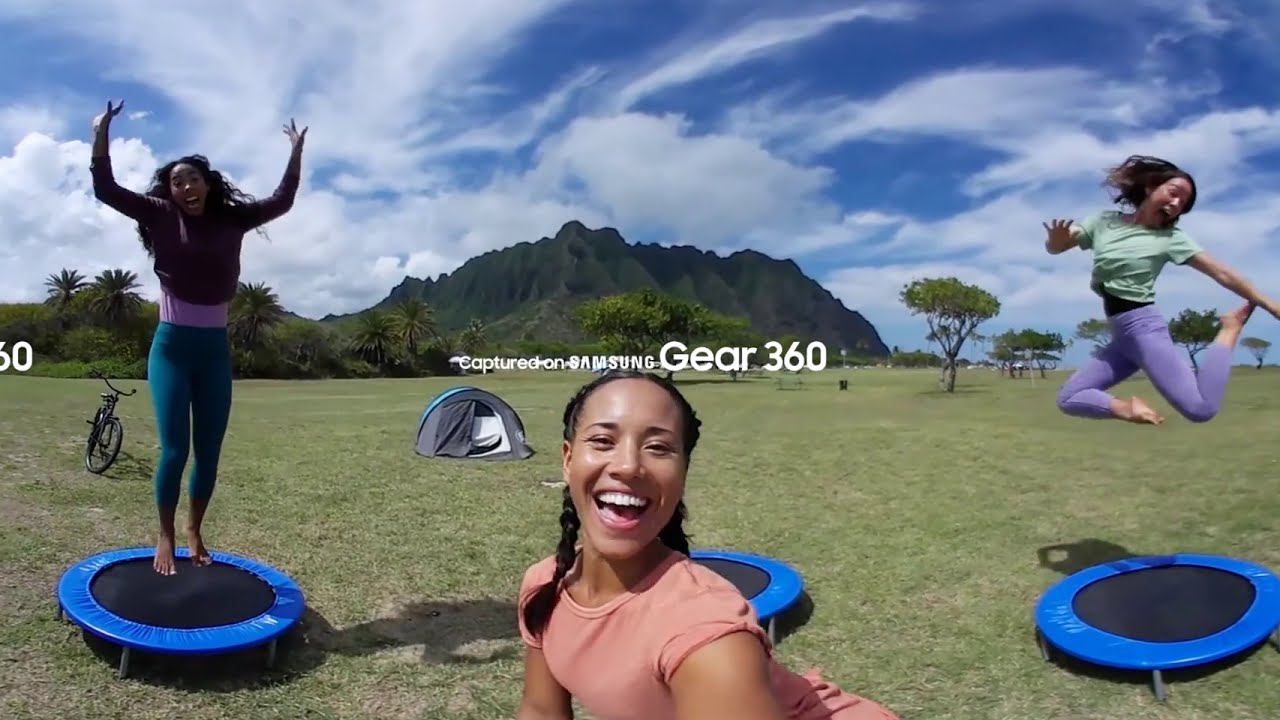In this vibrant outdoor setting, the image captures three women enjoying their time on trampolines, surrounded by lush greenery, and set against the backdrop of a distant green mountain. The scene appears tropical, possibly near an ocean. At the far back of the image, numerous trees stand in front of the mountain, painting a picturesque background.

In the foreground, a woman with long pigtails, dark braided hair, and a smile graces the center of the image. She wears a peach short-sleeved T-shirt and holds the camera, which has a watermark reading "Captured on Samsung Gear 360" prominently displayed in the middle. Close behind her are three small, blue-and-black trampolines.

On the left trampoline, a woman with dark hair, dressed in turquoise leggings and a purple top, leaps barefoot with arms raised, her joy evident. There is a bike parked to her left. To the right, another woman with purple leggings, a green shirt, and a dark undershirt jumps high, her hair flying wildly, and face etched with exuberance. The tent behind these trampolines features a grey front and blue top, dome-shaped and cozy-looking.

The entire scene exudes a sense of fun and energy against a sky filled with beautiful, fluffy white clouds and hints of blue. The trio appears to be thoroughly enjoying their day in this beautiful natural setting.